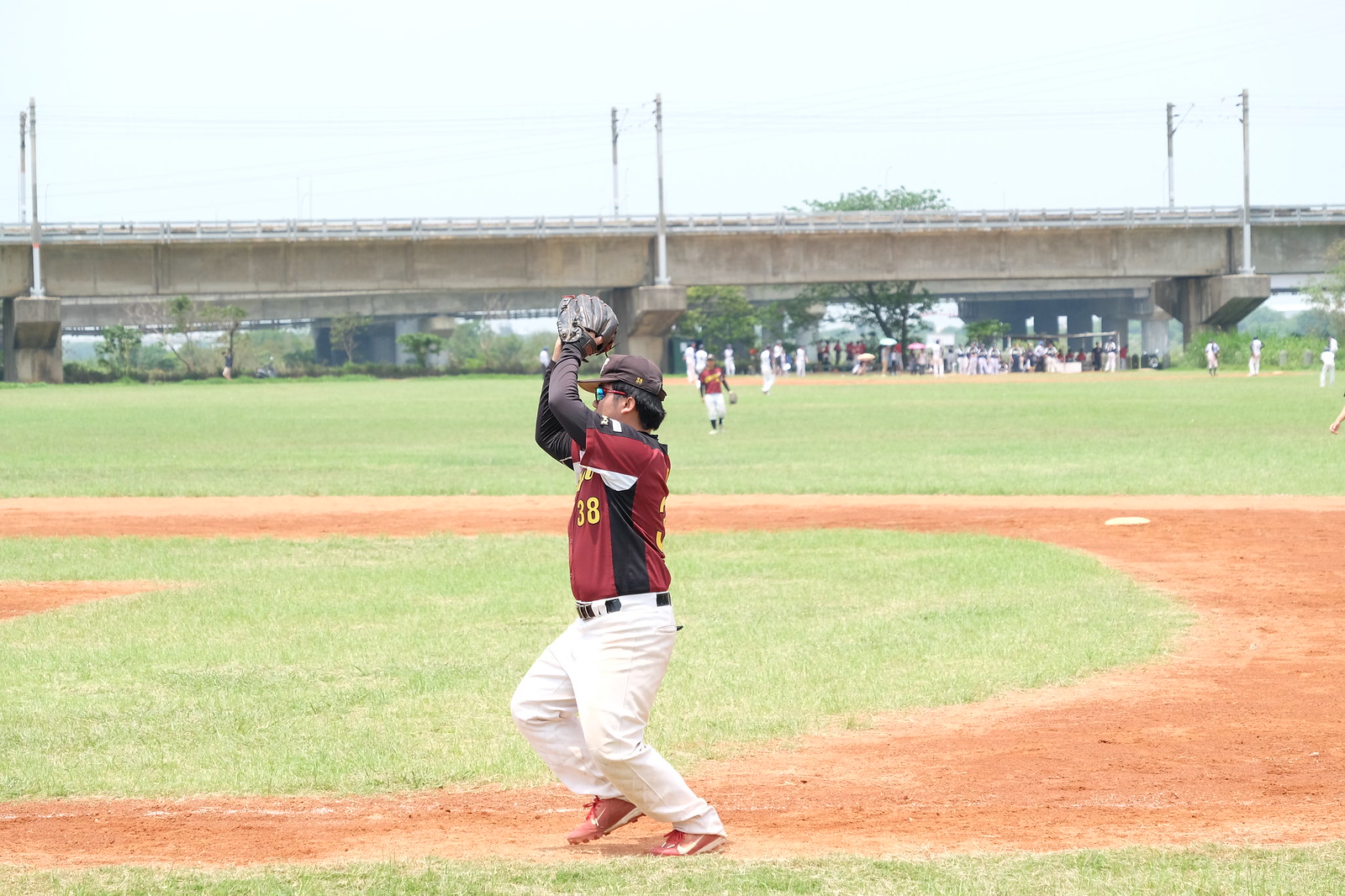The image captures a baseball game in progress, likely involving a local or minor league team, rather than professionals. The focal point is a player guarding first base, dressed in a distinctive maroon jersey with black stripes and yellow number 38 on the front. He wears a long black undershirt, white pants, red Nike cleats, and a black cap. Sunglasses cover his eyes, and his black glove is raised above his head, poised to catch an incoming ball. The brownish grass of the field extends to the green outfield, where another player in similar attire is visible. Spectators or perhaps another game can be seen in the distance. Dominating the background is a sizable, gray concrete bridge, adding to the local, unpolished charm of the scene. The sky remains clear in the upper portion of the image, providing a serene backdrop.